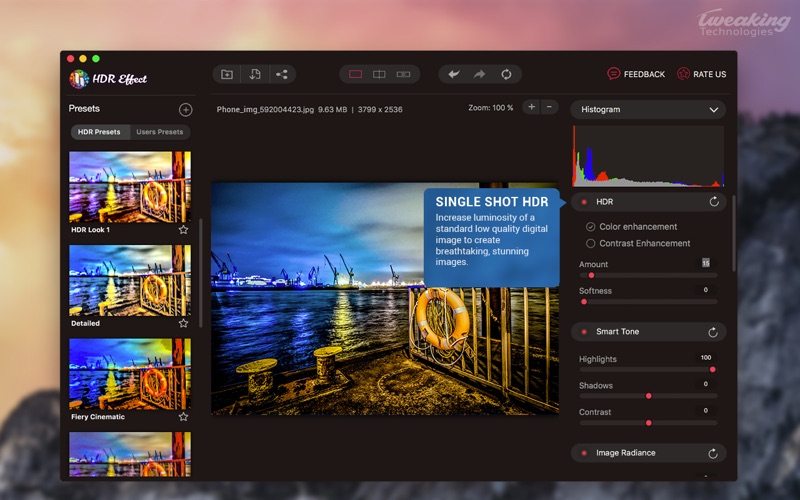The image showcases the back screen of a Mac displaying a photo editing software interface. The desktop background features a visually striking image resembling rocks. The software window is black and prominently displays the text "HDR effect," alongside several icons labeled "Feedback" and "Rate Us."

Within the software interface, a sidebar lists various presets divided into categories: "HDR Presets," "User Presets," with specific options such as "HDR Look 1," "Detailed," "Fiery," and "Cinematic." 

Central to the screen is a detailed graphic of a harbor or bay, which is predominantly blue. The image includes elements like a life buoy and ropes in the foreground, adding depth and context. 

Adjacent to the graphic, additional editing tools are visible, including sections titled "Histogram," "HDR," "Color Enhancement," "Contrast Enhancement," as well as sliders for adjusting "Amount" and "Softness." Further below, there are controls for "Smart Tone," "Highlights," "Shadows," "Contrast," and "Image Radiance."

The text "Single Shot HDR" indicates that the editing software specializes in HDR (High Dynamic Range) processing. Overall, the interface suggests a comprehensive and detailed photo editing environment tailored for enhancing images with HDR effects.